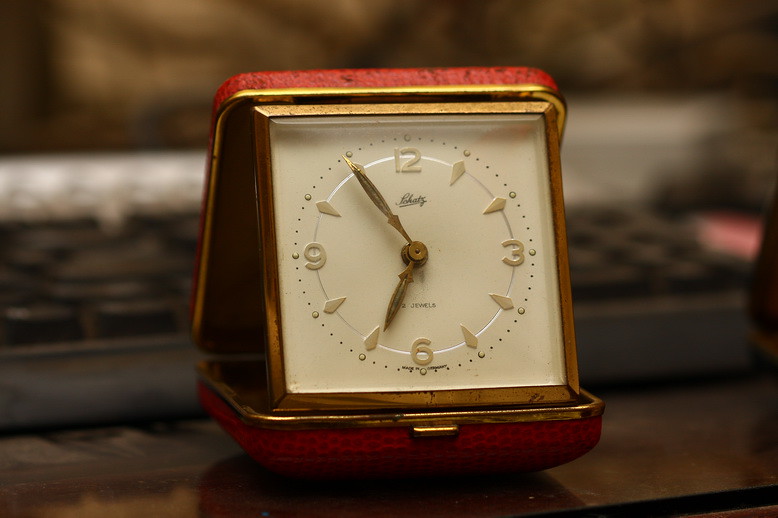This close-up photograph captures an old-fashioned portable travel clock positioned on a wooden surface. The clock, encased in a red foldable case that can snap shut, has a white square face with goldish-brown hands showing the time as 6:55. The numbers 12, 3, 6, and 9 are marked in light brown gold, with diamond-shaped dashes indicating the other hours. The face of the clock is surrounded by a gold-colored rim, and there's an italicized inscription "LOCAT" beneath the number 12, signifying the brand, along with "2 JOULES" above the number 6, partially obscured by the hour hand. The red case features a metal gold button that facilitates opening and closing. In the blurred background, there appears to be a black QWERTY keyboard, though the surrounding elements are indistinct. This vintage timepiece, designed for both display and portability, retains a classic charm.